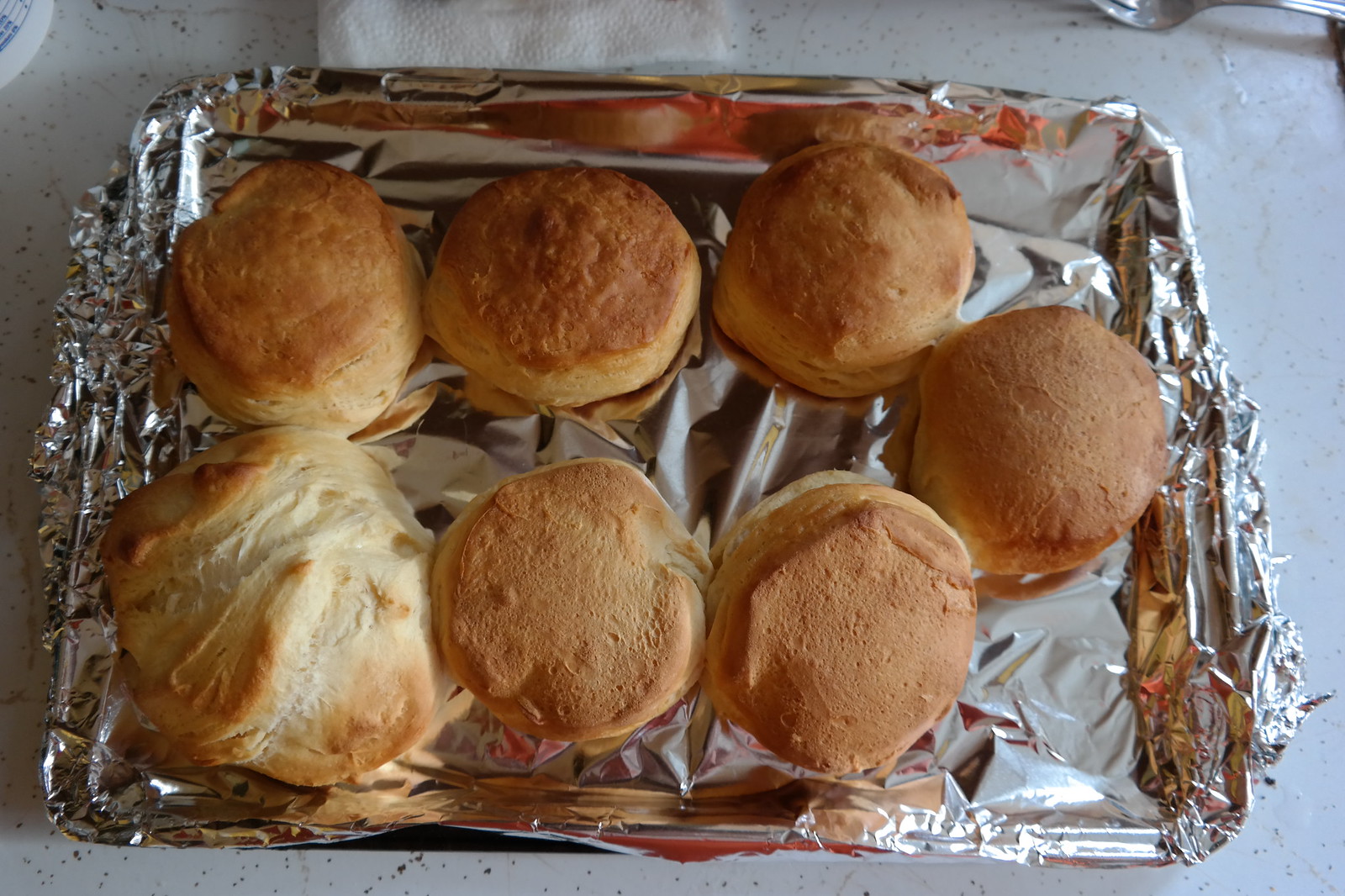This detailed image captures a close-up, downward shot of a baking sheet, covered with shiny aluminum foil, sitting on a white countertop with black speckles. On the tray are seven freshly baked biscuits, six of which are uniform in size and shape, with a golden-brown, toasty appearance. These biscuits look somewhat dry, with no butter or additional toppings applied. On the bottom left corner of the tray, there is an unusual, much larger biscuit. This bigger biscuit appears irregular in shape, almost as though it might be two biscuits that merged together during baking. It stands out from the rest due to its lighter color, with white patches indicating that it's not fully browned, suggesting it may not be completely cooked.